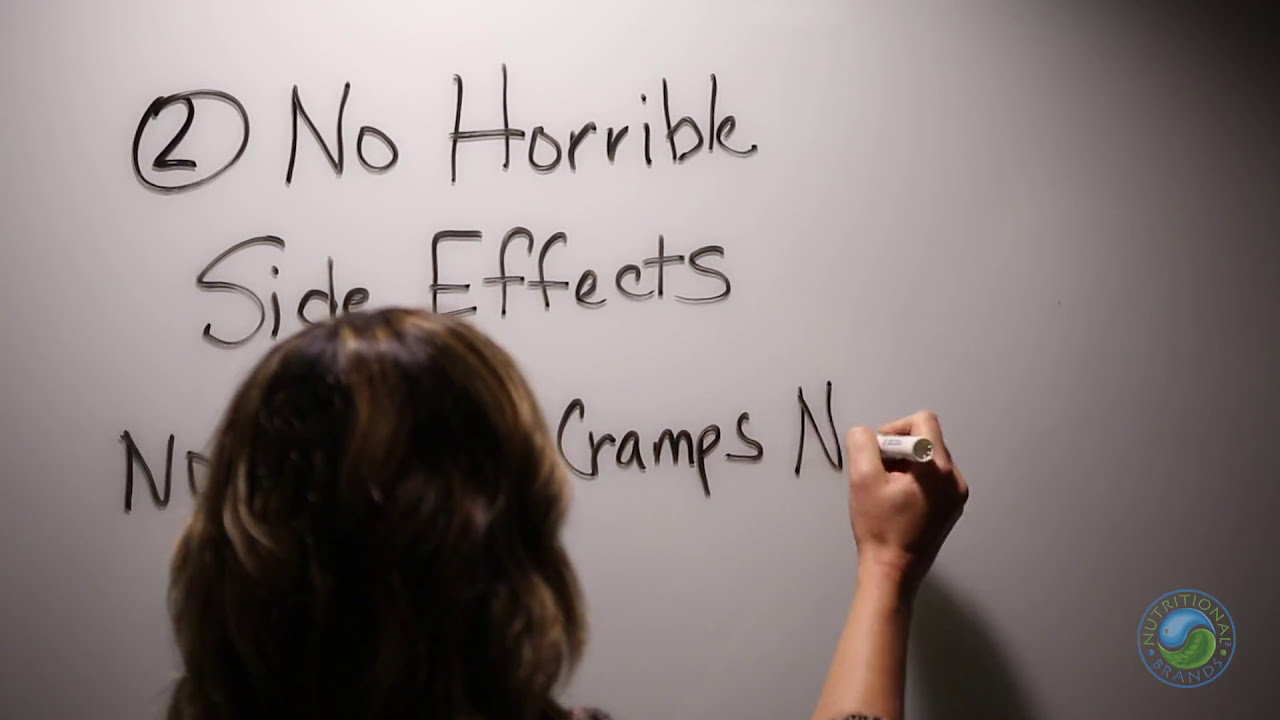The image features the back of a person with brown hair, possibly female, writing on a whiteboard. The scene is slightly blurry with a vignette effect, creating darker edges around the central focus. The person is using their right hand to hold a white-bodied dry erase marker with a black tip, actively writing on the board. The whiteboard contains text that begins with a circled number "2," followed by the phrases "No horrible side effects" and "No [obscured] cramps," with further text obscured by the person's head. The background includes a logo in the bottom right corner that reads "Nutritional Brands," encircled by a blue and green yin-yang symbol. The logo suggests affiliation with a health or wellness company.